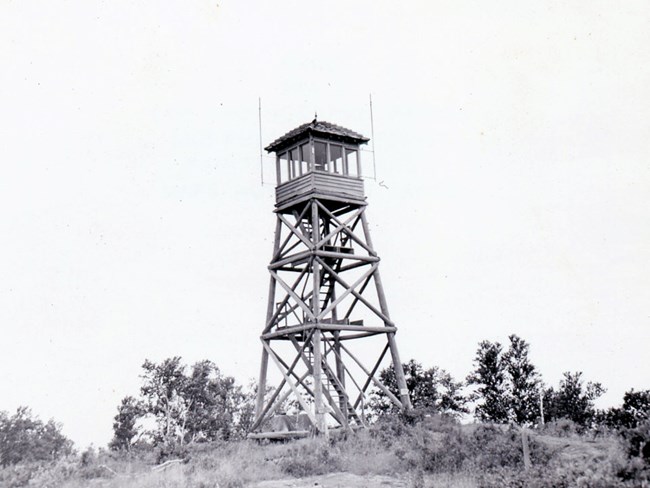This black and white photograph captures a fire watch tower perched atop a hillside, surrounded by various trees, bushes, and dirt hills in the foreground. The tower, constructed from a combination of wood and steel, zigzags upward with three sets of stairs leading to a wooden and glass-enclosed top. This upper section features multiple windows, a shingled roof, and two thin, small radio antennas protruding from its sides. The overall structure appears to be four stories high. The sky dominates the background, appearing either cloudy or completely clear, though its exact state is indeterminate due to the black and white nature of the image. A trapdoor is also visible, providing access to the watch cabin where observers can monitor for fires.